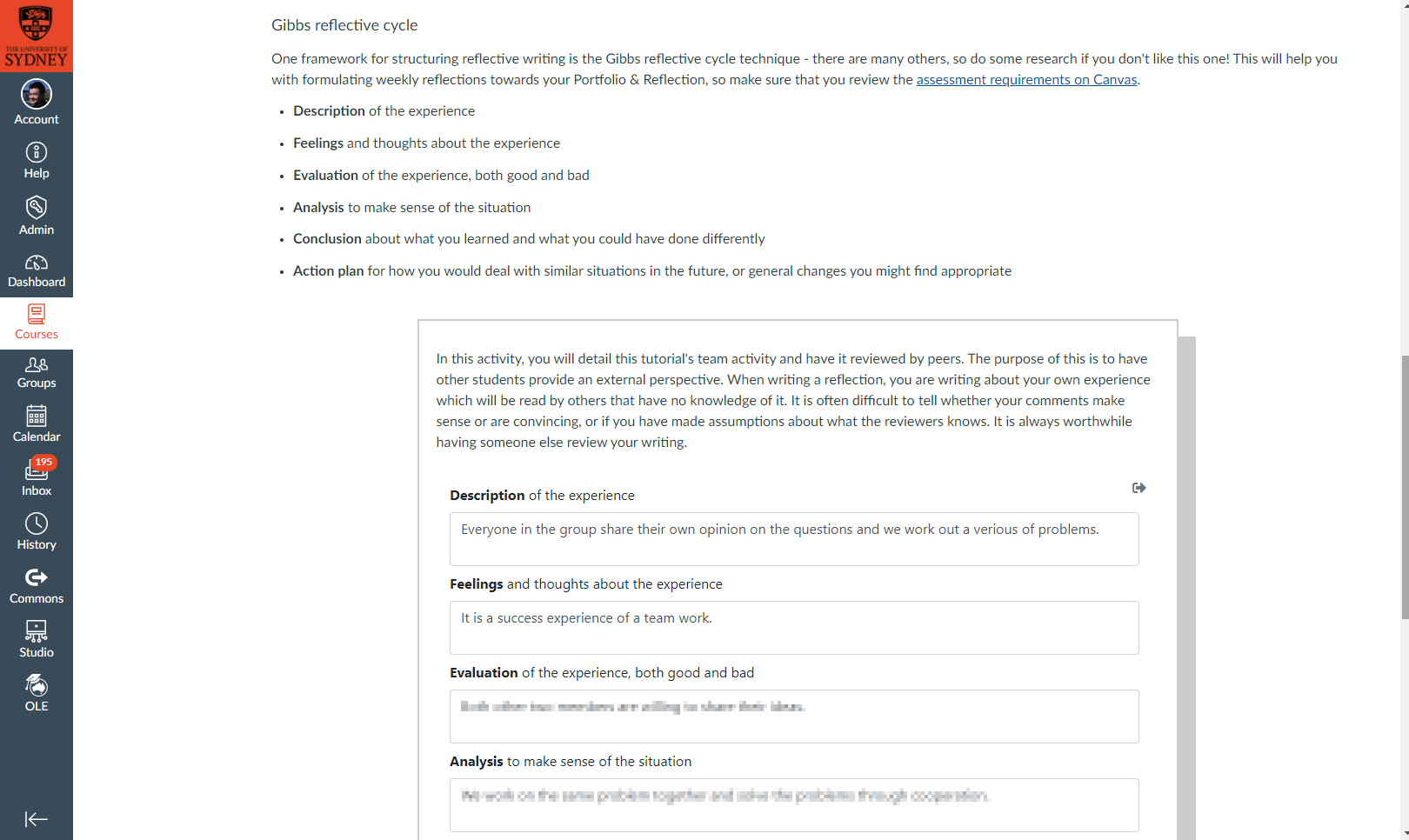![Gibbs Reflective Cycle Instructions - University of Sydney]

The image is a screenshot from an educational platform associated with the University of Sydney. On the left-hand side, there is a vertical gray border featuring a red section at the top with the University of Sydney's name and coat-of-arms-style icon. Below this, a menu lists various options: Account, Help, Admin, Dashboard, Courses, Groups, Calendar, Inbox, History, Commons, Studio, and OLE, with "Courses" highlighted in white.

On the right-hand side, set against a white background, the text explains Gibbs Reflective Cycle, a framework for structuring reflective writing. It suggests researching other frameworks if Gibbs is not suitable. The instructions emphasize the importance of weekly reflections for portfolio development and meeting assessment criteria on Canvas. The reflection structure includes:

1. Description of the experience.
2. Feelings and thoughts about the experience.
3. Evaluation of the experience, both good and bad.
4. Analysis to make sense of the situation.
5. Conclusion about lessons learned and potential improvements.
6. Action plan for handling similar situations in the future or suggesting relevant changes.

Students are instructed to detail their tutorial team's activities and have their reflections reviewed by peers for external perspectives. This peer review aims to ensure clarity and effectiveness in conveying individual experiences to readers unfamiliar with the specific situations.

Text boxes are provided for: 
- Description of the experience
- Feelings and thoughts about the experience
- Evaluation of the experience, both good and bad
- Analysis to make sense of the situation